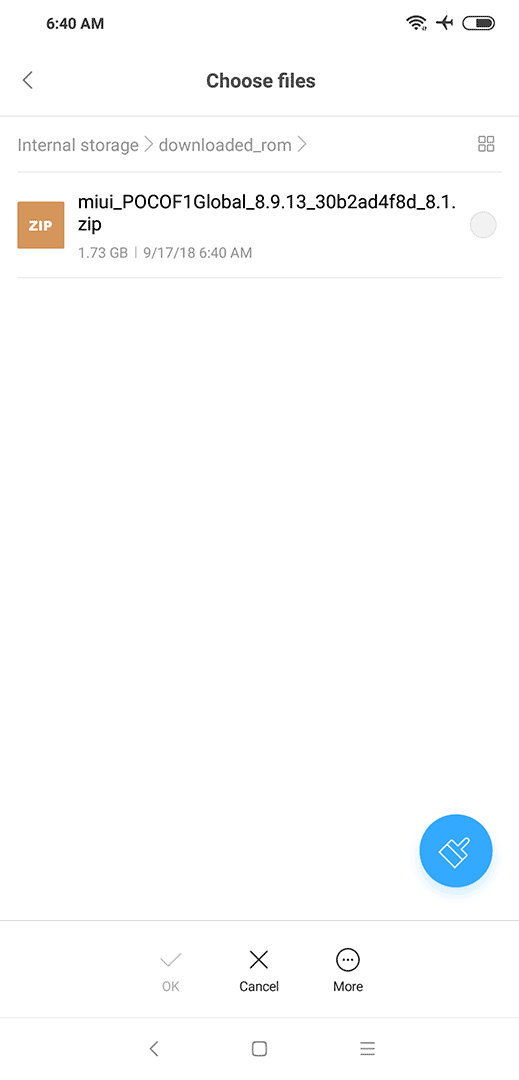The screenshot captured from a cell phone displays an interface at 6:40 a.m. The phone is in airplane mode with Wi-Fi connected at full strength and the battery approximately half-charged, as indicated in the upper right corner of the screen.

Below the status indicators, there is a navigation bar featuring a back arrow on the left. Centrally located is the text "Choose files" in bold black font. Underneath this, there is a pathway that reads "Internal storage" followed by a right-pointing arrow, "downloaded_ROM" followed by another right-pointing arrow, and a grid icon with four small squares forming a larger square on the right side.

Beneath this pathway, an orange box labeled "zip" in white letters is displayed. Next to it, a file named "MIUI_POCOF1_global_8.9.13_30B2AD4F8D_8.1.zip" is shown. This file is marked with a bullet point that is not highlighted. Additional details about the file are provided below, stating its size is 1.373 gigabytes and it was last modified on September 17, 2018, at 6:40 a.m.

In the lower right corner, there is a blue circle featuring a paintbrush icon. Below this section, there are three action options: "OK" accompanied by a check mark, "Cancel" with an X mark, and "More" with a circle and three dots.

At the bottom of the screen are the standard navigation buttons: a back button, a home button, and a toggle applications button.